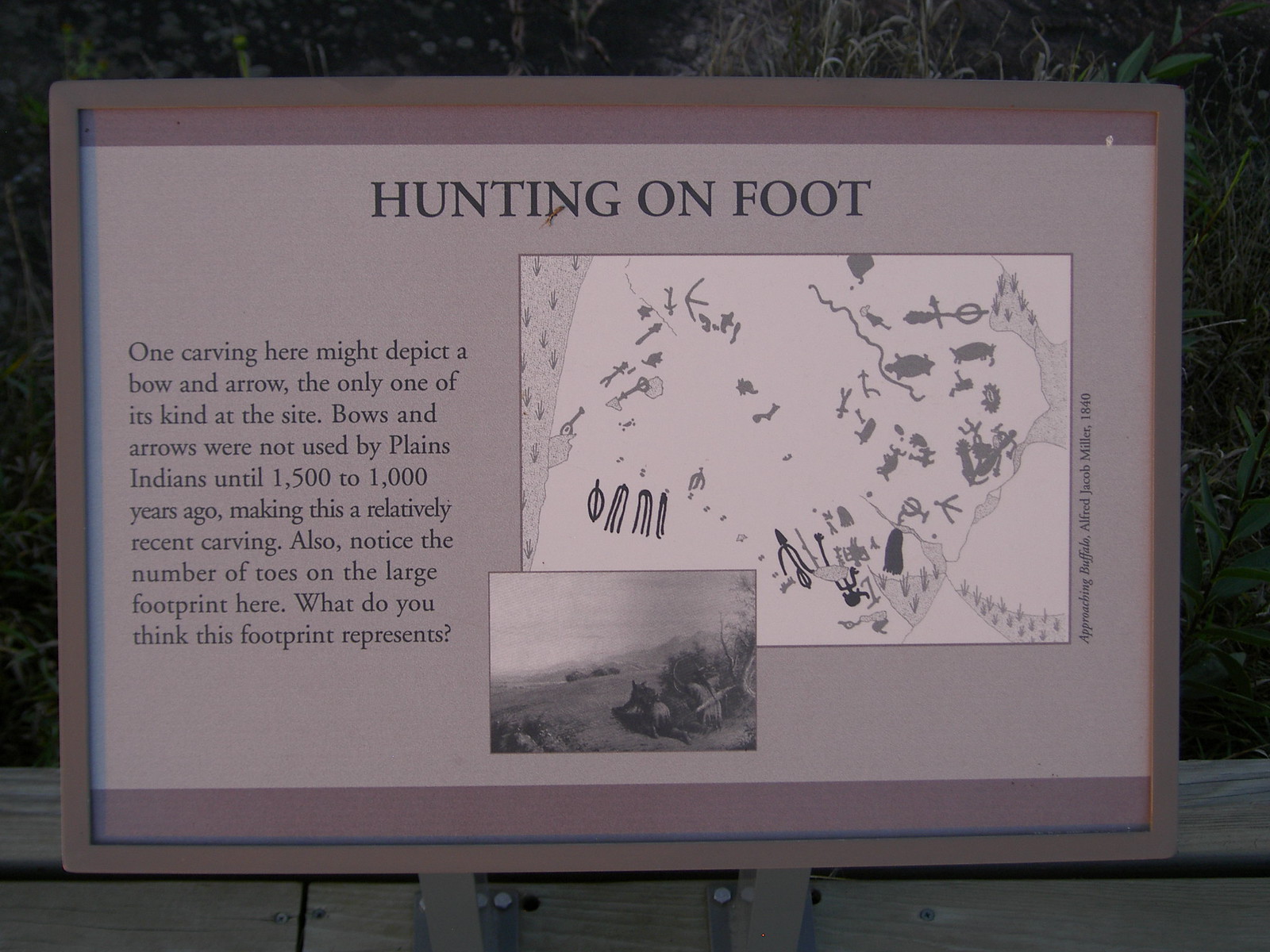The image shows a detailed informational plaque, likely located at a zoo or along a hiking trail. The plaque is rectangular with a light gray background, bordered by a light gray frame and accented with rust-colored bands at the top and bottom. Dominating the center in large black font is the title "Hunting on Foot." Below the title, on the left side, text describes a unique carving that might depict a bow and arrow, noted as the only one of its kind at the site. This carving is significant because Plains Indians did not use bows and arrows until 1,500 to 1,000 years ago, making it a relatively recent addition. Attention is also drawn to a large footprint depicted on the plaque, with a prompt asking viewers to consider what the footprint might represent. On the right side of the plaque, there is a black-and-white map featuring 2D animal silhouettes, including a turtle at the top right and what appears to be a squirrel. Additionally, a smaller black-and-white image shows either a wolf or a dog in a field with a mountain range and sky in the background, further enriching the scenic narrative. Although some words to the right of the map are written sideways and difficult to read, the overall context provided is richly detailed and encourages interactive engagement with the depicted historical and natural elements.